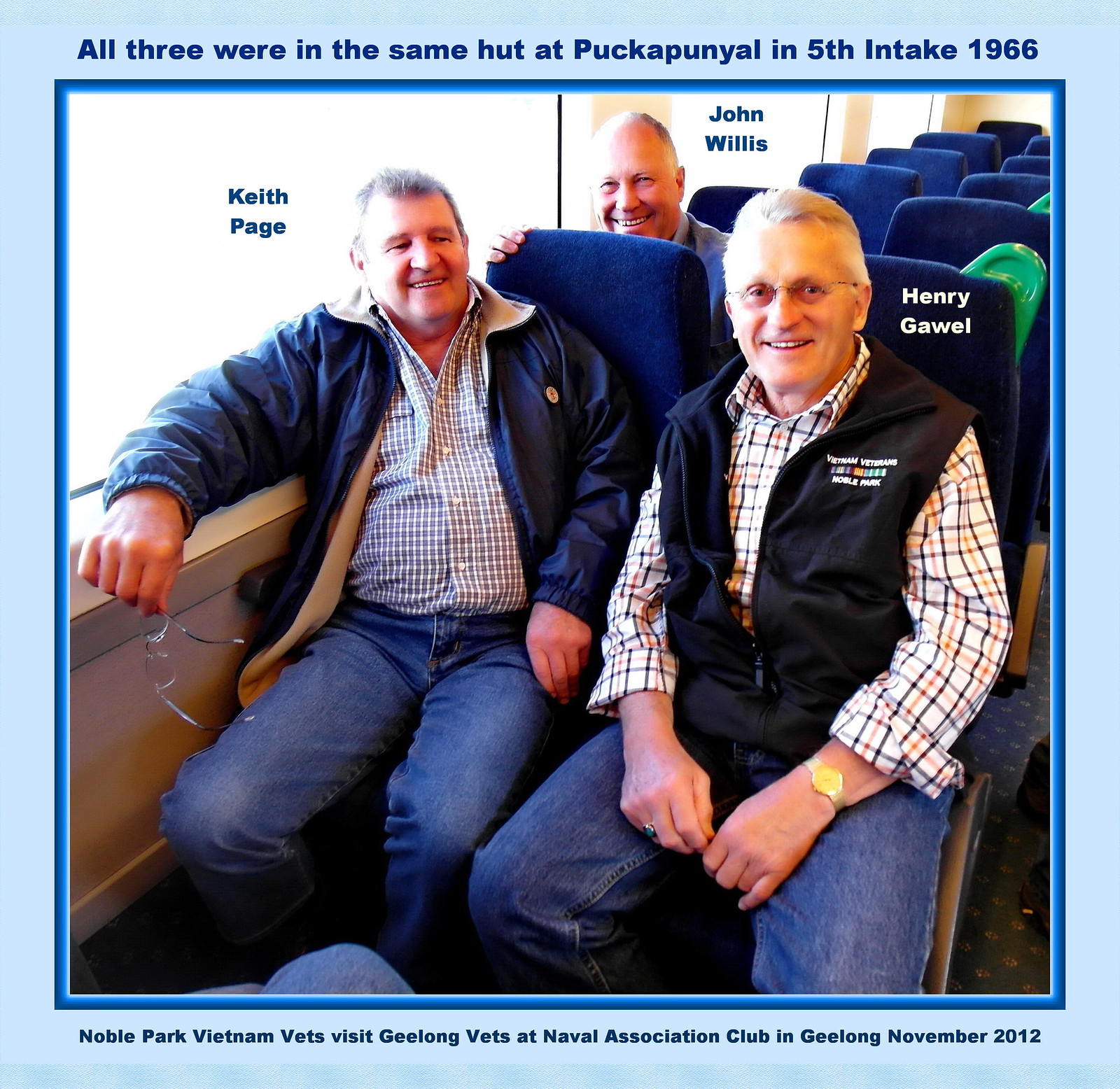This color photograph, bordered in blue, captures three Vietnam veterans seated in blue chairs, with text indicating their shared history and a recent reunion. Above the image, the text reads, "All three were in the same hut at Puckapunyal in the 5th Intake, 1966." Below, it states, "Noble Park Vietnam vets visit Geelong vets at Naval Association Club in Geelong, November 2012." The men, all looking directly at the camera and smiling, are identified by names next to their faces. Keith Page, on the left, wears a long-sleeved blue jacket over a checkered button-down shirt and blue jeans, holding his glasses in his right hand. To his right, Henry Gowell sports a checkered button-down shirt paired with blue jeans and a dark blue zip-up vest. Behind them, in the next row of chairs, John Willis is partially visible, donning a blue shirt. The setting appears reminiscent of a bus or train. The photograph commemorates the enduring bond formed during their military service and their continued camaraderie decades later.